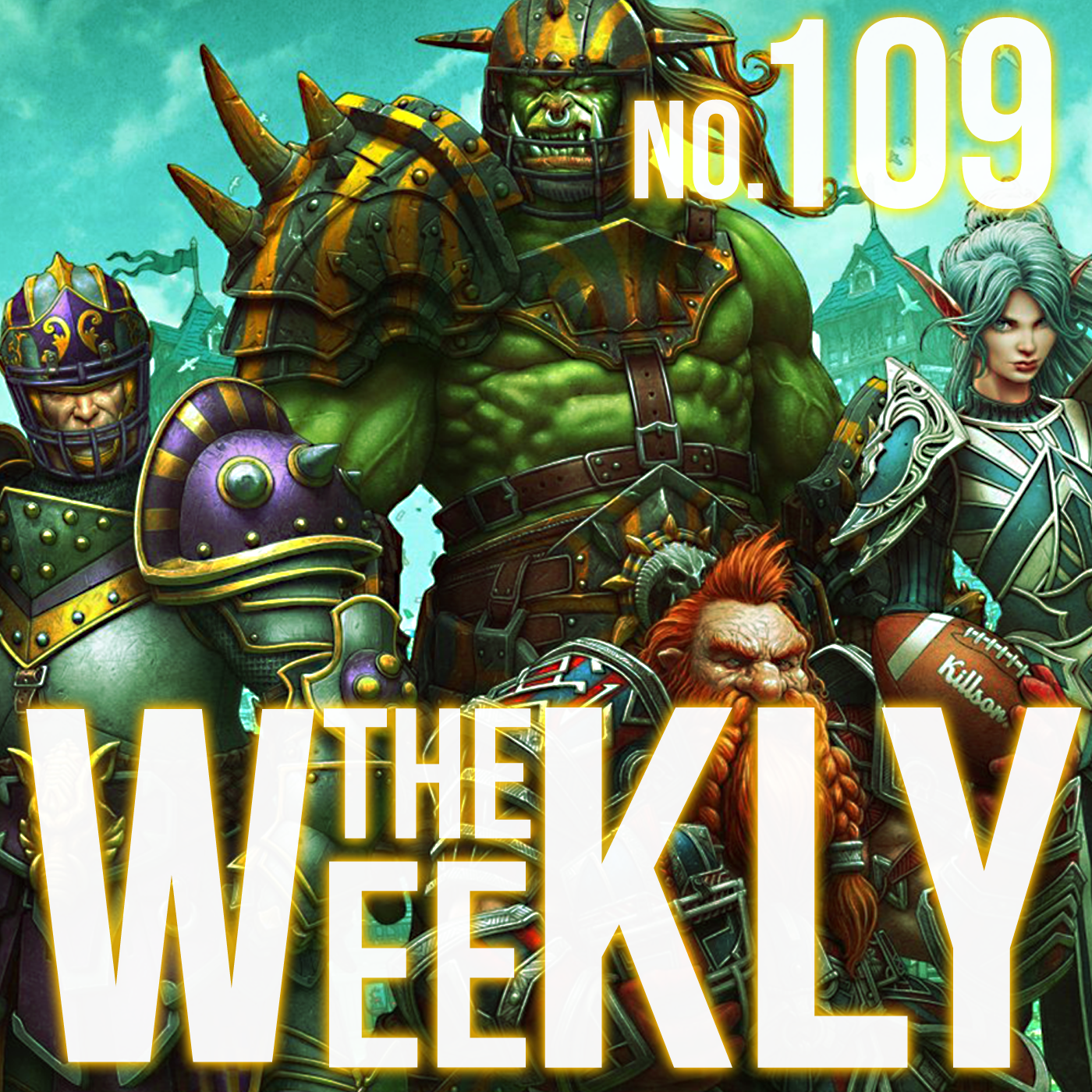In the image, set against a blue background with a partial view of a house, there are four detailed fantasy characters prominently featured. At the center is a large green orc-like figure resembling the Hulk, adorned in a helmet and spiked shoulder armor, with leather straps around his waist and torso. To his left stands a heavily armored knight in a purple and gold helmet. To his right is a serious-looking female character with light blue hair and matching light blue armor. Positioned at the bottom is a red-haired dwarf with a braided beard, holding a football labeled "Kilsin." The scene is framed with bold text, where "The Weekly" is written in white and outlined in yellow at the bottom, and the number 109 appears in the top right corner.